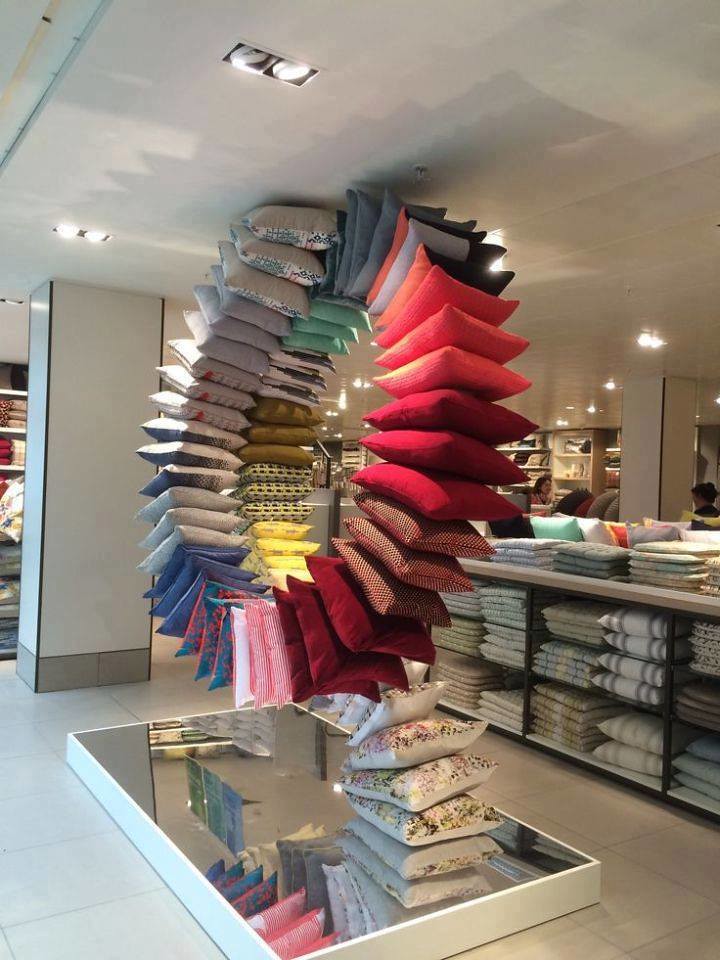The photograph captures the interior of a homeware store, showcasing an impressively intricate and eye-catching display. At the center of the image is a dramatic, large wreath-like loop of cushions, possibly three to four feet in height, suspended in mid-air. These cushions create a visually engaging doughnut shape that both draws attention and allows a view through its center to the rest of the store. The array of cushions, mounted likely on an unseen pole, spans a spectrum of colors including reds, corals, mauves, pinks, whites, slates, and even patterned designs, arranged in a spiraling or fan-like formation.

The base of the display features a reflective mirror, further highlighting the multitude of cushions, some of which are also placed on the ground. The backdrop consists of organized shelving units holding neatly folded blankets of various styles and colors, displayed in cubbyholes and on top surfaces. A vertical column typical in commercial settings supports the roof structure, while the large white ceramic tiled flooring, with darker gray grout lines running diagonally, provides a clean, contrasting foundation for the vivid display.

The ambient lighting is soft and unobtrusive, with recessed can lighting in the ceiling casting an even illumination that enhances the vibrancy of the colorful pillows against the otherwise neutral store decor. The overall aesthetic is one of meticulous organization blended with creative flair, making for a truly neat and memorable retail display.